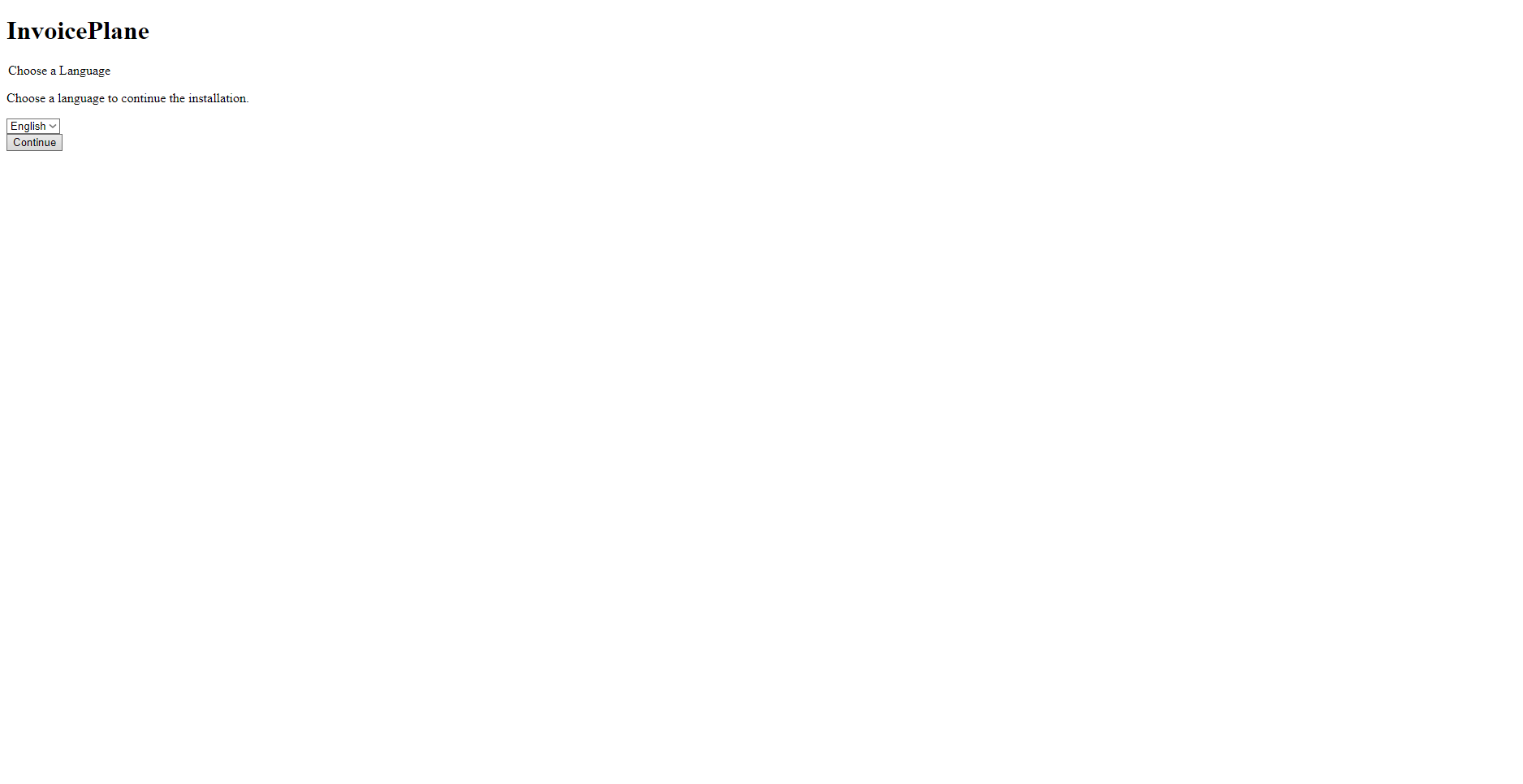The screenshot displays an almost entirely blank white page, except for some text and a few user interface elements at the top left. The most prominent feature is the title in bold black text reading "Invoice Plane," indicating the name of the software. Directly below, in much smaller black text, is the instruction "Choose a language," followed by an explanatory line that reads "Choose a language to continue the installation." Beneath these lines, there is a dropdown menu defaulting to "English," presumably offering other language options such as Spanish, Chinese, and Russian. Below the dropdown menu, there is a button to proceed with the installation process after selecting the desired language. The layout and text suggest that this is the preliminary setup screen for an invoicing software program designed to help manage and send invoices to businesses or customers.